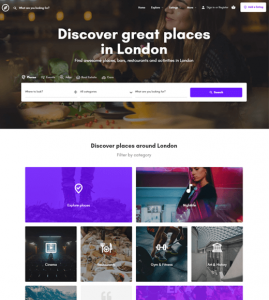This image showcases a landing page for a travel website specializing in flight itineraries. Dominating the top third of the page is a large header featuring a vibrant background photograph of a woman in a restaurant, surrounded by an array of appetizing foods. Overlaying this image is a bold, white text that reads, "Discover Great Places in London." Below this text is a white bar containing search filters for destination and other options, although some details are unclear. A prominent purple search button is located on the right side of the bar.

Just beneath the main header is a section titled "Discover Places Around London," which is visually represented by six individual photographs. The first image on the left is distinguished by a purple hue and features a check mark. The second image depicts a woman, possibly enjoying music through headphones. The next four images highlight various activities and attractions: a cinema, culinary experiences, exercise opportunities, and museums.